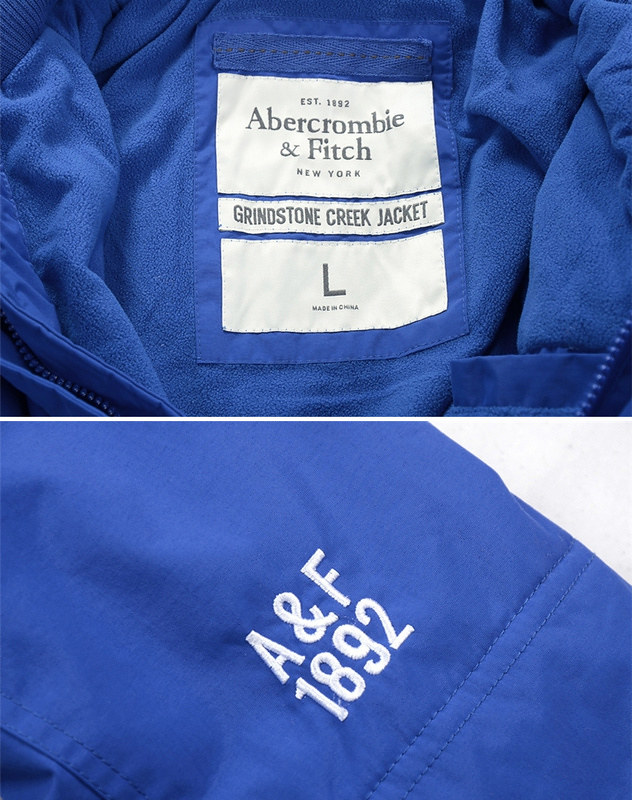The image appears to be a composite of two separate photos. The bottom half of the image features a red jacket with a white monogram that reads "A&F 1892." The top half showcases the inner part of a blue jacket, which has a label with various inscriptions. The label reads "EST 1892 Abercrombie & Fitch, New York, Grindstone Creek Jackets" in black text, and underneath it, it indicates the size "L" for large and notes that the garment is made in China. The blue jacket, as noted from the label, extends to the zipper and continues to exhibit the same blue color throughout.